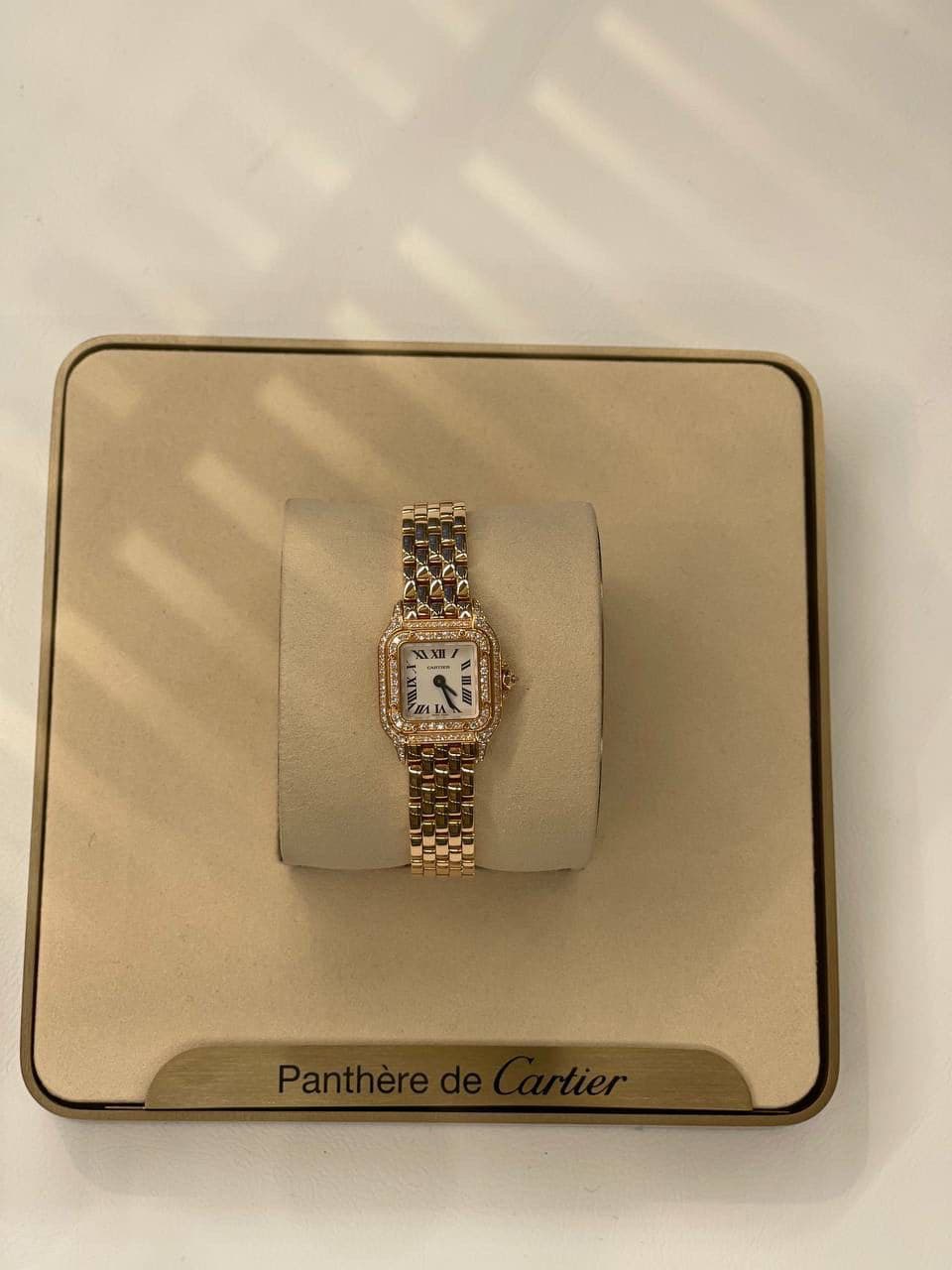This photograph showcases a luxurious gold Panthère de Cartier watch displayed in its original packaging. The watch features a fully golden, expandable wristband and a square face with black Roman numerals encircling the dial. The gold bezel appears to be adorned with tiny gems or is exceptionally shiny, contributing to its elegant aura. Positioned on a beige, circular holder, the watch exhibits an hour and a minute hand set against a gleaming white face. The display is resting on a cardboard stand within a beige display case, all set atop a pristine white table. Below the watch, a golden plaque reads "Panthère de Cartier" in black lettering. The overall presentation, combined with the untouched and gleaming quality of the watch, suggests that it is brand new and has never been worn. Subtle reflections and shadows hint at light passing through a window or grate above, enhancing the watch's exquisite detail and craftsmanship.